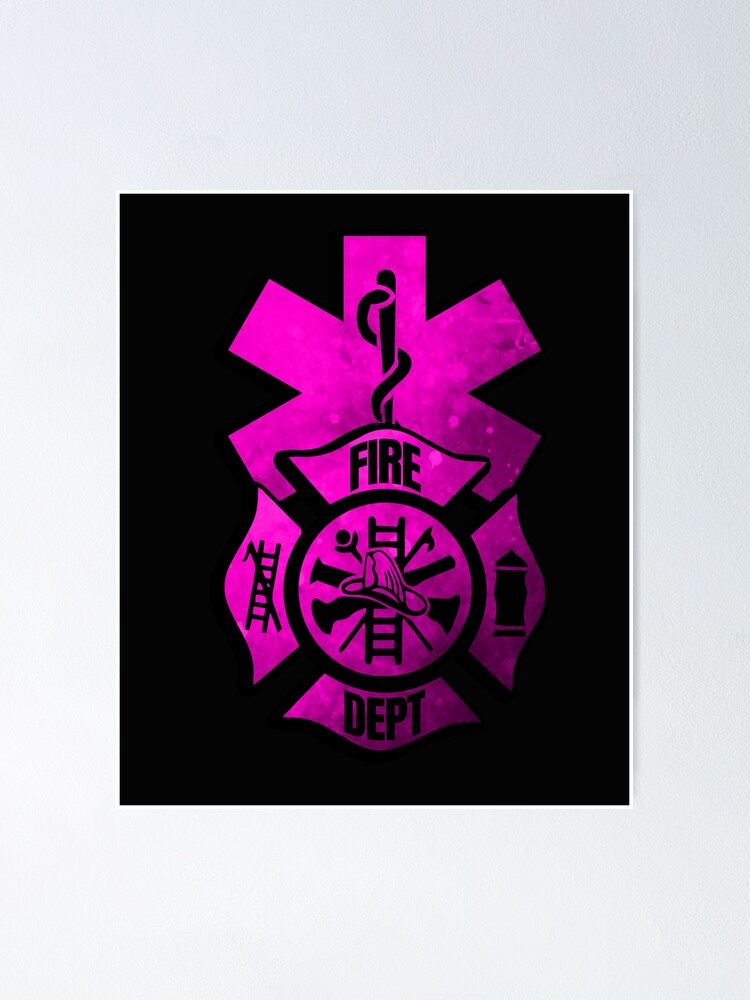The image displays a detailed and symbolic firefighter's emblem set against a black background. The emblem itself features a predominantly purple hue, with intricate elements and symbols in shades of black and purple. At the top of the badge, a purple Maltese cross is adorned with a black pole entwined by a snake, a reference to the EMT symbol. Surrounding a central circle, the top arm of the cross features the word "FIRE" while the bottom arm spells out "DEPT." The central circle showcases essential firefighting tools, including a firefighter's helmet, a ladder, and an axe, all intricately drawn and overlapping. To the left of the circle, another ladder is accompanied by a crowbar, while the right side features a detailed fire hydrant. The emblem, a long-standing symbol of gallantry, perseverance, loyalty, and protection, is a testament to the profession's rich heritage and commitment.